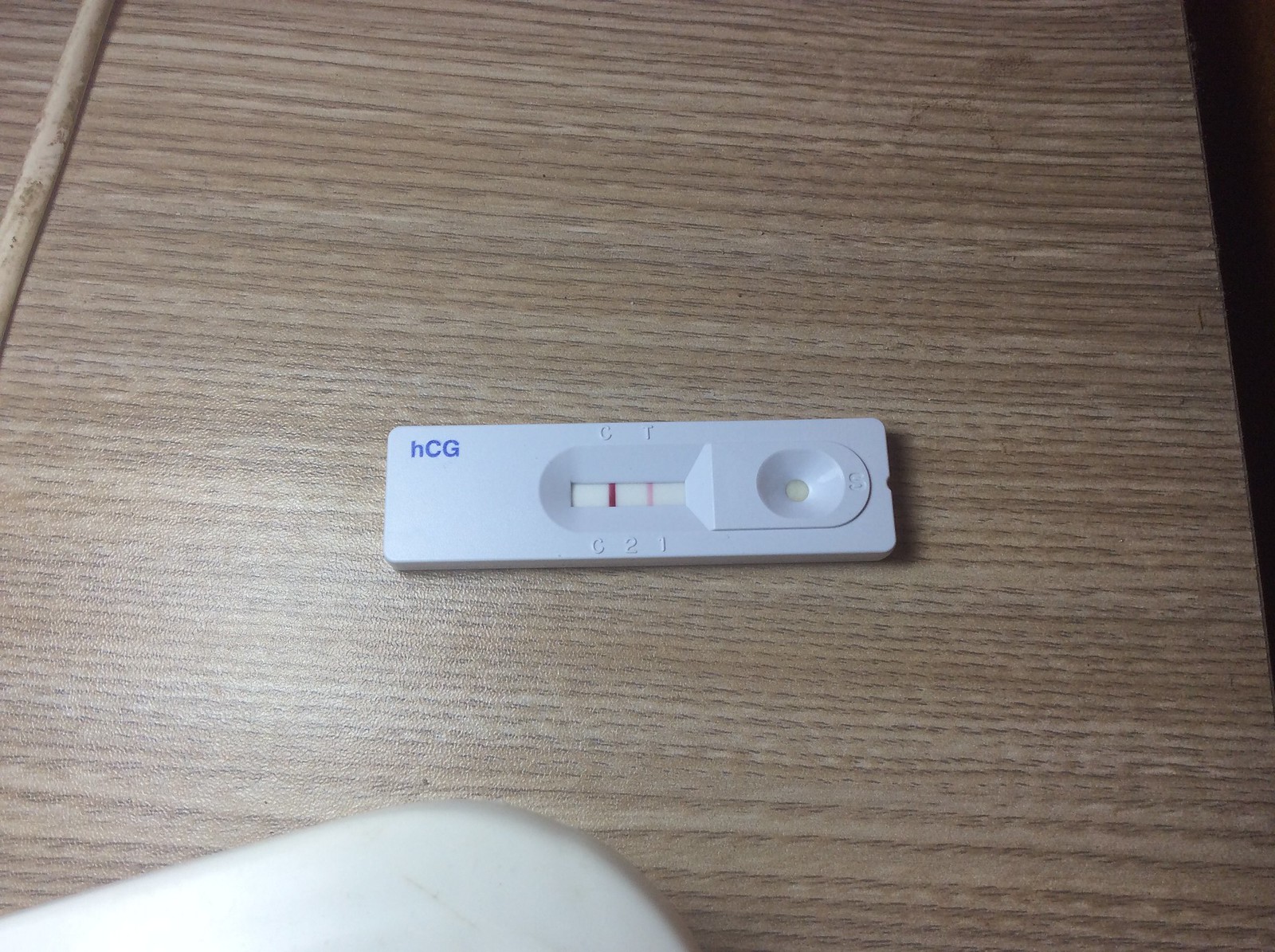This photograph, presented in landscape orientation, prominently features a rectangular medical test device, which appears to be a pregnancy test. The device is positioned horizontally, with its width extending from the left to the right side of the image. In the upper left-hand corner of the test, the letters "hCG" are printed, signifying its intended use for detecting the hormone associated with pregnancy.

The test device appears to have been used, as indicated by two vertical bands visible near the top: a dark red band aligning with the embossed letter "C" and a faint pink band above the embossed letter "T." There is a small recessed area on the right side of the device, likely meant for placing a urine sample.

Further details include additional embossed lettering towards the bottom of the device, marking "C," "2," and "T." The entire pregnancy test rests on a surface with a noticeable wood grain texture, running horizontally from left to right. An out-of-focus, whitish object is also visible in the lower left-hand part of the image, but its identity remains unclear.